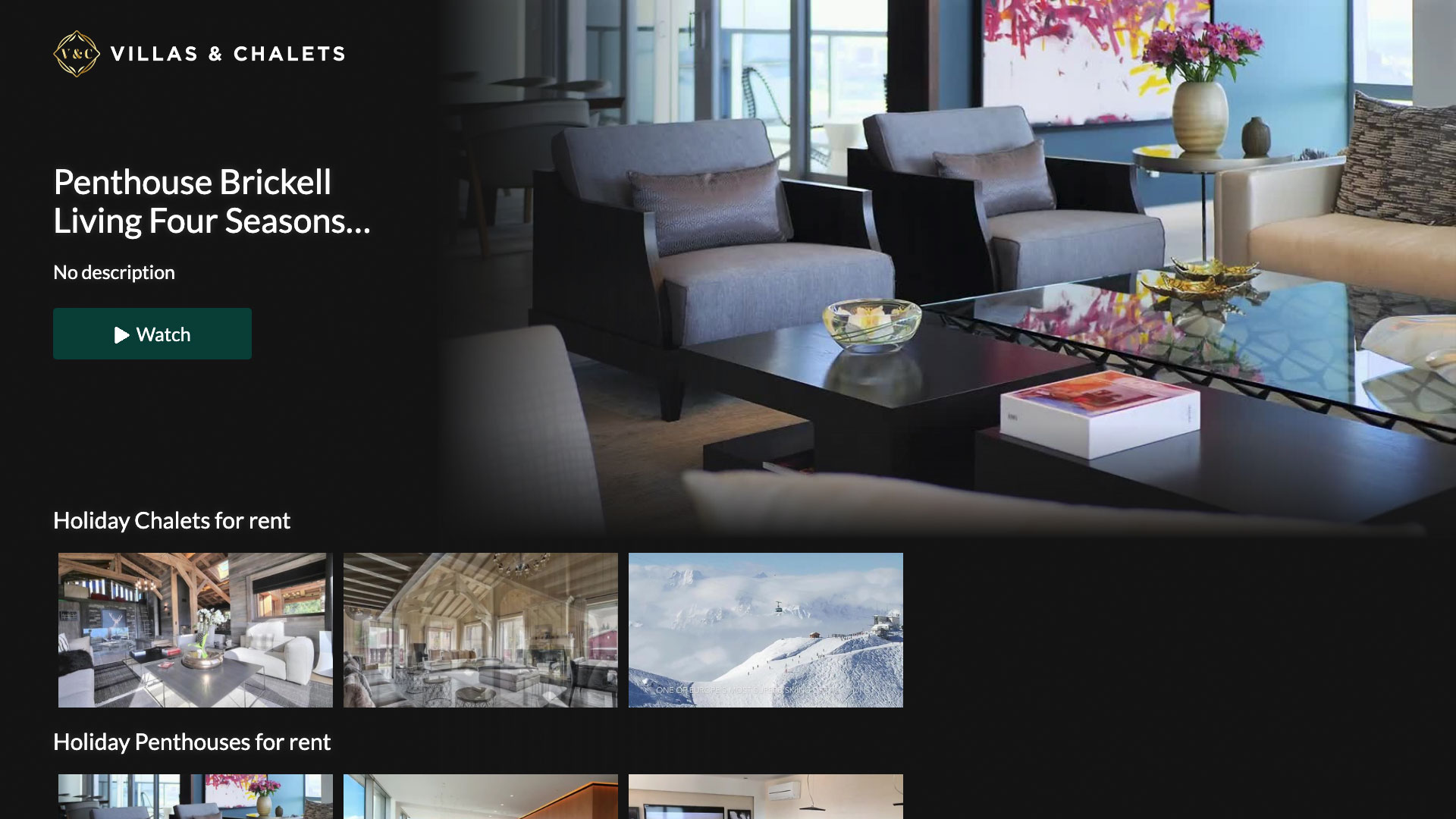**Detailed Descriptive Caption:**

The image is a screenshot from a real estate website, captured at the very top of the webpage. On the upper left, the header lists various categories in bold text: “Villas and Chalets.” Directly beneath this header, additional categories are partially visible, including “Penthouse, Brickell, Living, Four Seasons,” followed by an ellipsis indicating more text that is not visible in the screenshot. 

Underneath this, there is a notable message saying "No description," which likely refers to missing or incomplete information. Below this message is a prominent green button labeled "Watch on the Inside," inviting users to view interior details, possibly through a video or virtual tour.

Further down the webpage, there is a section titled "Holiday Chalets for Rent," showcasing a series of thumbnail images depicting various holiday homes or buildings available for rental. These images are organized to give a visual representation of the available properties.

Subsequent to this section, there is another one titled "Holiday Penthouses for Rent." Although the section is partially cut off, it displays more thumbnail images of additional properties, indicating an extensive listing beyond what is fully visible in the screenshot.

Positioned centrally on the page is a larger image, likely a feature image, showing an elegant lobby area. This central image could be representative of the quality and style of the properties listed on the site.